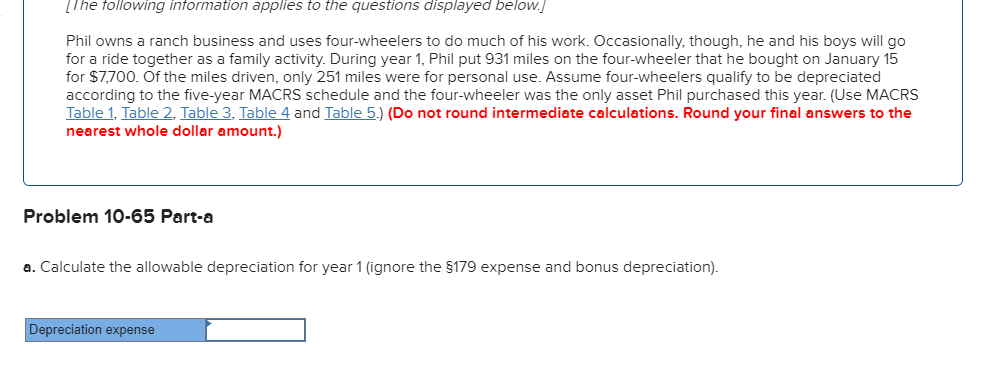This image displays a detailed story problem, likely part of a homework assignment or examination on accounting or tax depreciation. At the top, a box contains contextual information relevant to the questions below. It mentions that Phil owns a ranch business where he uses four-wheelers for work-related purposes. Sometimes, Phil and his sons use the four-wheelers for family activities. During the first year, Phil accumulated 931 miles on a four-wheeler he purchased on January 15th for $7,700. Out of these, 251 miles were for personal use. The problem states that four-wheelers qualify for a five-year MACRS (Modified Accelerated Cost Recovery System) depreciation schedule and notes that this is the only asset Phil acquired that year. The instructions point to using MACRS Table 1 through Table 5 for calculations, specifying not to round intermediate calculations but to round the final answers to the nearest whole dollar. This specific part of the problem, labeled as "Problem 10-65 Part A," asks to calculate the allowable depreciation for the first year, ignoring the $179 expense and bonus depreciation.